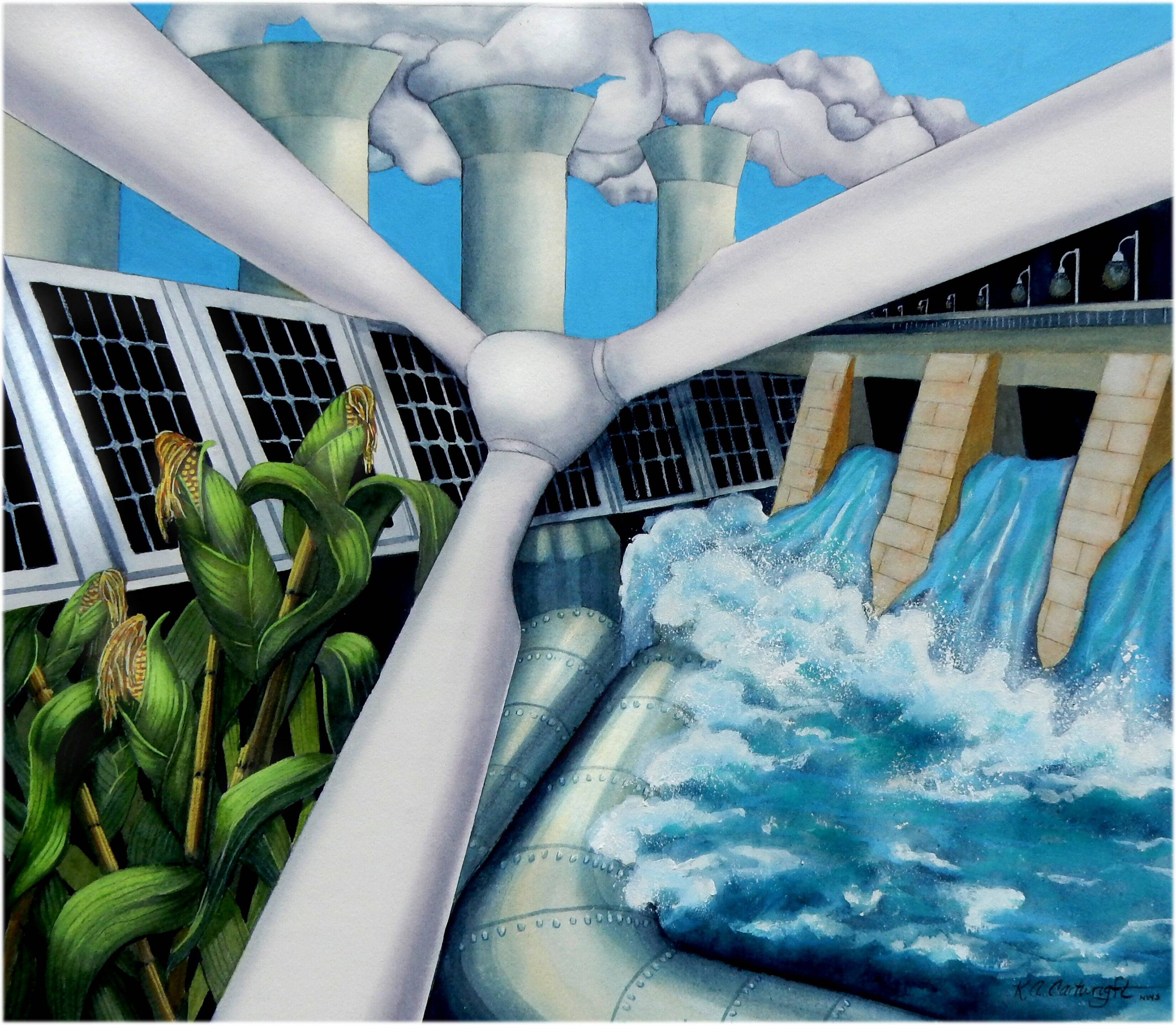The image is a detailed artwork with a theme likely related to global warming or renewable energy. Horizontally aligned and rectangular, the top fourth features an almost clear blue sky with four tall, cylindrical smoke stacks that widen at the top, emitting billowing white clouds of smoke or steam drifting to the right. The shadow of the stacks falls on their left side.

Dominating the center foreground is a large, white windmill with gray-shaded blades. The windmill's hub is rounded, with one blade pointing to the upper left, one to the edge, and another descending to the left. The light appears to emanate from the center-left of the image, creating subtle shadows.

Between the windmill and the smokestacks is a row of seven solar panels arranged in a grid pattern, each with a silver or gray frame and a black background divided into smaller squares. Some additional solar panels lie beneath the windmill blades near the hub.

In the upper right, a light gray raised highway supported by tan brick pillars emerges, creating diagonal shadows and featuring streetlights. Beneath the highway, water flows and pools, framed by white waves and foam. This water management system is contained by metal panels, likely screwed together, with another set of panels to their left.

On the lower left, large ears of corn with green leaves and corn silk grow, positioned within the triangular area formed by the windmill blades.

This intricate image, possibly a public service announcement, juxtaposes various renewable energy sources like wind, solar, and hydro power against the backdrop of industrial smokestacks, weaving together elements of environmental consciousness and technological advancement.